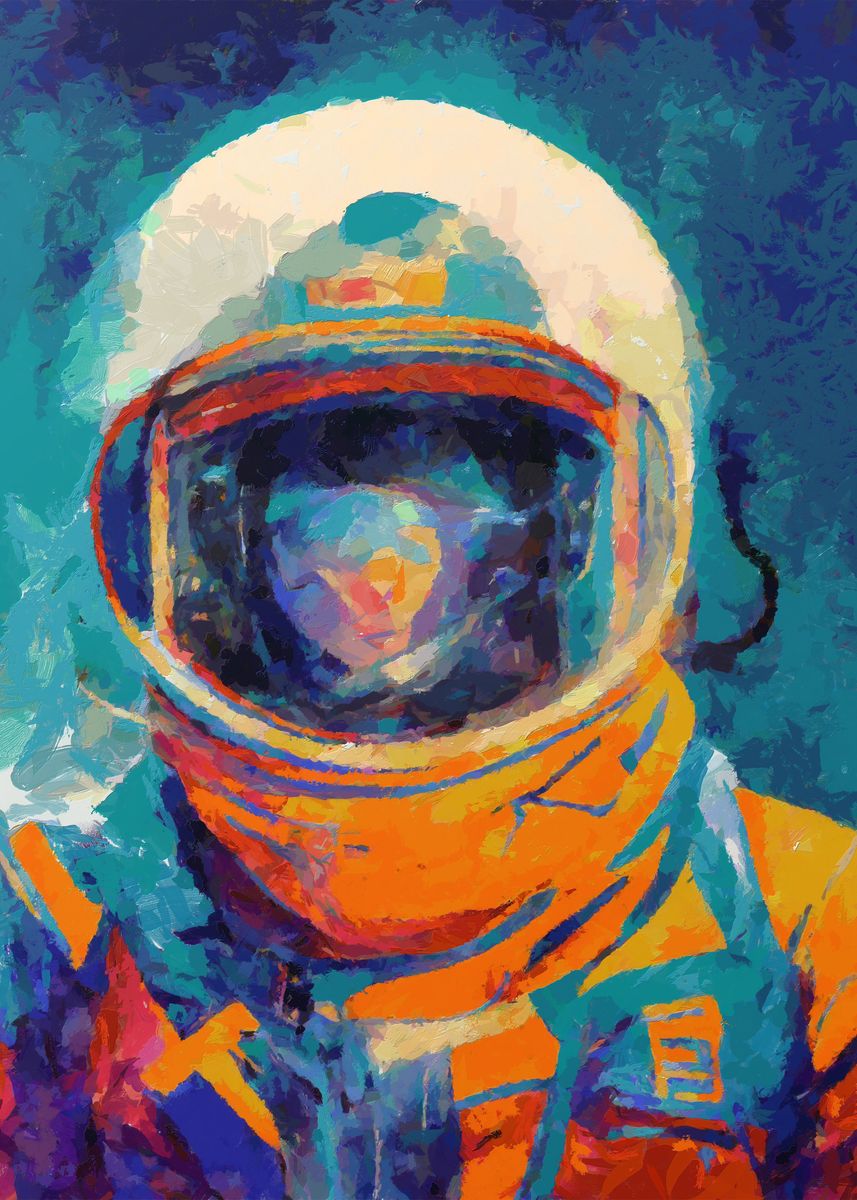This artwork is a highly stylized painting, possibly an oil painting, depicting an astronaut in a brightly colored spacesuit. The suit is dominantly orange with blue accents, including a black cord running from the helmet to the suit, and various pockets and straps adorning the shoulders. The astronaut is wearing a helmet with a large, clear visor, featuring reflections that suggest the image of a woman with long hair, though no skin or direct facial features are visible. The background transitions from cyan to dark blue, creating a gradient effect that complements the astronaut figure and adds depth to the painting. The composition is focused from the astronaut’s chest to slightly above the head, with the helmet itself being white with additional orange detailing. Heavy brush strokes emphasize the artistic, dynamic feel of the image.